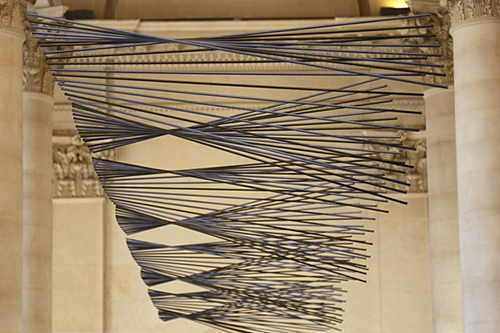This photograph captures an intricately designed courtyard featuring prominently arranged stone columns with ornate carvings at their tops. These columns, appearing to be a mix of white and beige hues, create a structured pathway. Stretching horizontally across the columns are interwoven strands, which seem to be a mix of blue and brown materials or sticks, creating an elaborate crisscross pattern. These strands form X shapes and straight lines, contributing to a visually captivating ceiling cover that enhances the courtyard's architecture. The background reveals a further extension of the rustic columns against a yellowish-beige ceiling, adding depth and cohesion to the scene.